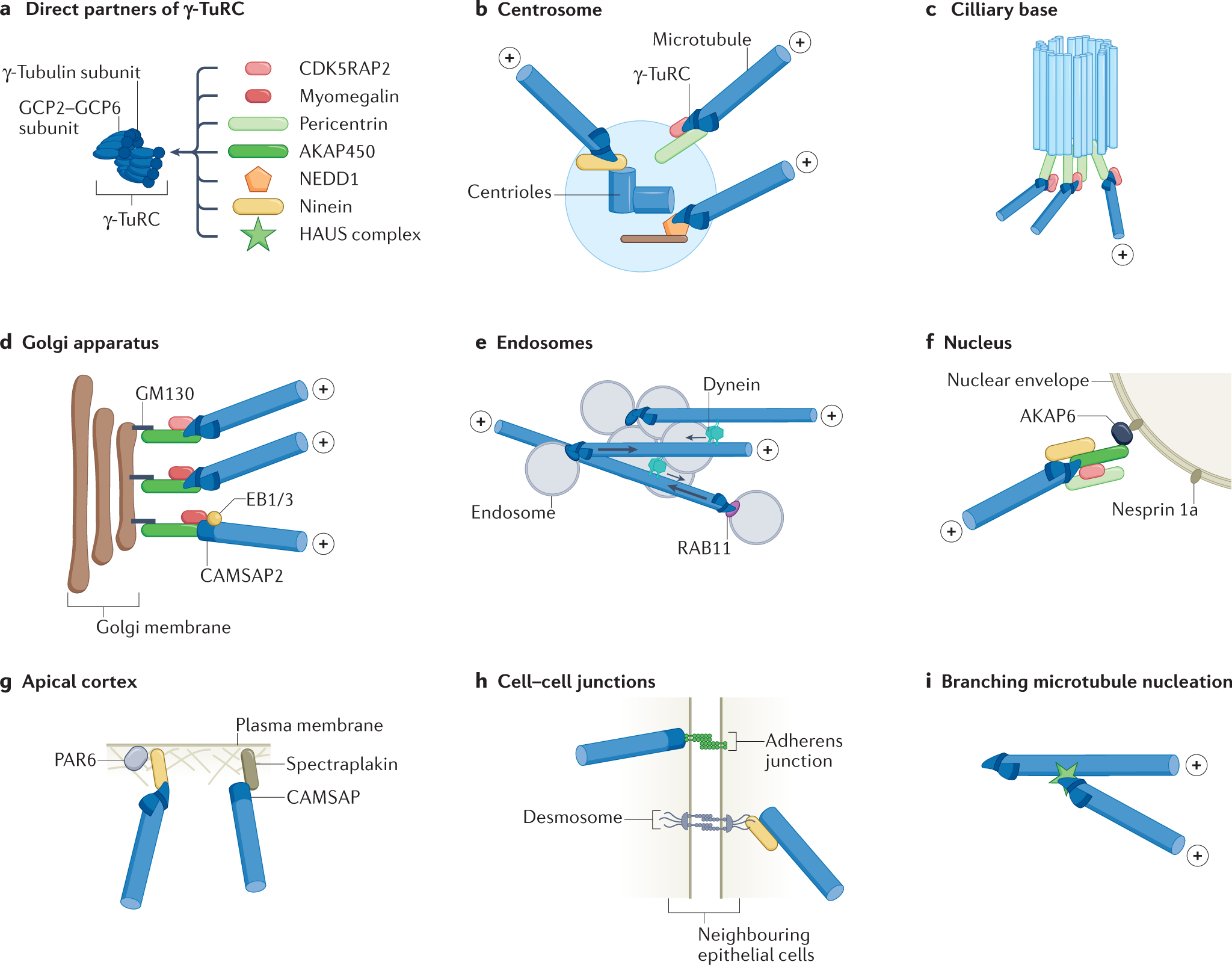This detailed image is an educational diagram likely sourced from a textbook or instructional material, depicting the organized structure and various components of a cell, color-coded for clarity. The diagram consists of nine labeled illustrations, arranged from A to I. 

- **A**: A color-coded chart depicting the **direct partners of Y-TURC**. The chart features colors such as pink, red, light green, dark green, orange, yellow, and multiple shades of green, with black text on the right for annotations.
- **B**: Illustrates the **centrosome**, showing the microtubule organization center.
- **C**: Represents the **ciliary base**, crucial for the formation and function of cilia.
- **D**: Displays the **Golgi apparatus**, involved in protein and lipid modification and transport.
- **E**: Shows **endosomes**, which are involved in transporting and sorting cellular material.
- **F**: Highlights the **nucleus**, the control center of the cell containing genetic material.
- **G**: Indicates the **apical cortex**, associated with the cell's structural polarity.
- **H**: Depicts **cell-cell junctions**, showing connectivity and communication points between cells.
- **I**: Illustrates **branching microtubule nucleation**, showing the formation of microtubules at various branching points.

The central image of the diagram features blue tubulin subunits intersecting with labels pointing to various components, illustrating the intricate and interconnected nature of cellular structures. The entire diagram includes technical terms and detailed labeling to aid in the understanding of each cellular component's function and relationship.